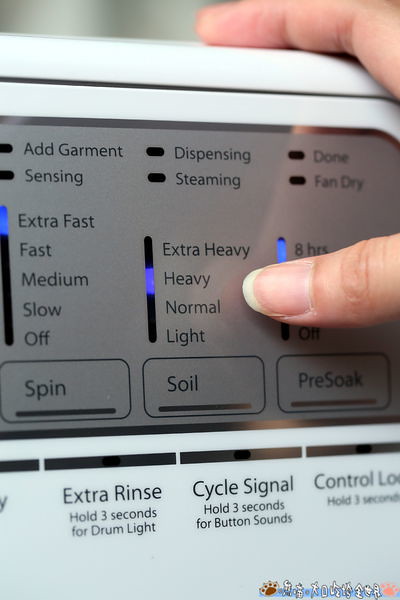A detailed close-up photograph features the control panel of a washing machine, mainly white with a gray digital interface. At the top right edge, a person's thumb and finger are seen pressing on the controls. The control panel itself is divided into multiple sections. At the very top, there's a thin white line going across from left to right, followed by a gray section containing two rows of three items: "Add Garment," "Sensing," "Dispensing," "Steaming," "Done," and "Fan Dry." Below these, there are three vertical sliding bars used for various settings: "Spin" with options "Extra Fast," "Fast," "Medium," "Slow," and "Off"; "Soil" with choices "Extra Heavy," "Heavy," "Normal," and "Light"; and "Pre-Soak" with an option labeled "Eight Hours."

Further down, below the sliding bars, are additional controls: "Extra Rinse," "Cycle Signal," and "Control Lock," each with instructions like "Hold 3 Seconds for Drum Light," "Hold 3 Seconds for Button Sounds," and a partially obscured control on the far right. The rightmost edge of the panel features some blurred text and a silver glitter detail in the bottom right corner.